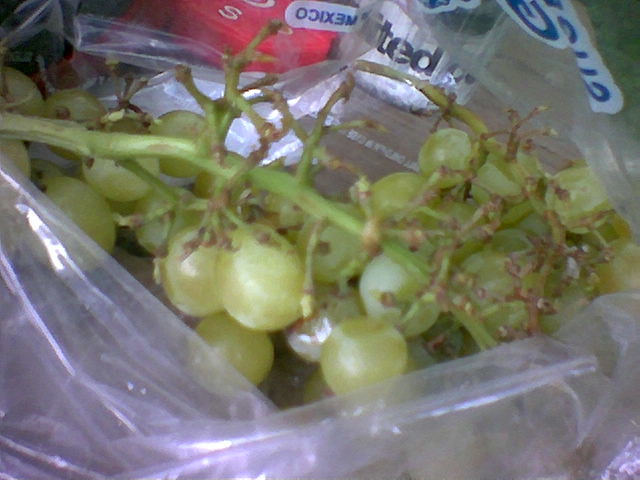This is a close-up photograph of a bag of seedless green grapes. The grapes are contained in a clear plastic display bag, with the text "Mexico" visible in the distance on the plastic—though the text appears reversed. The grapes themselves vary in color, with several being a light yellow-green, suggesting uneven ripeness and some appear overripe. The grape stems are green, but many branches are bare, indicating that some grapes have already been picked off. In the background, there are indistinct shapes, likely including a water bottle and two soda cans, slightly out of focus. The overall image is of marginal quality, emphasizing the texture and condition of the grapes.